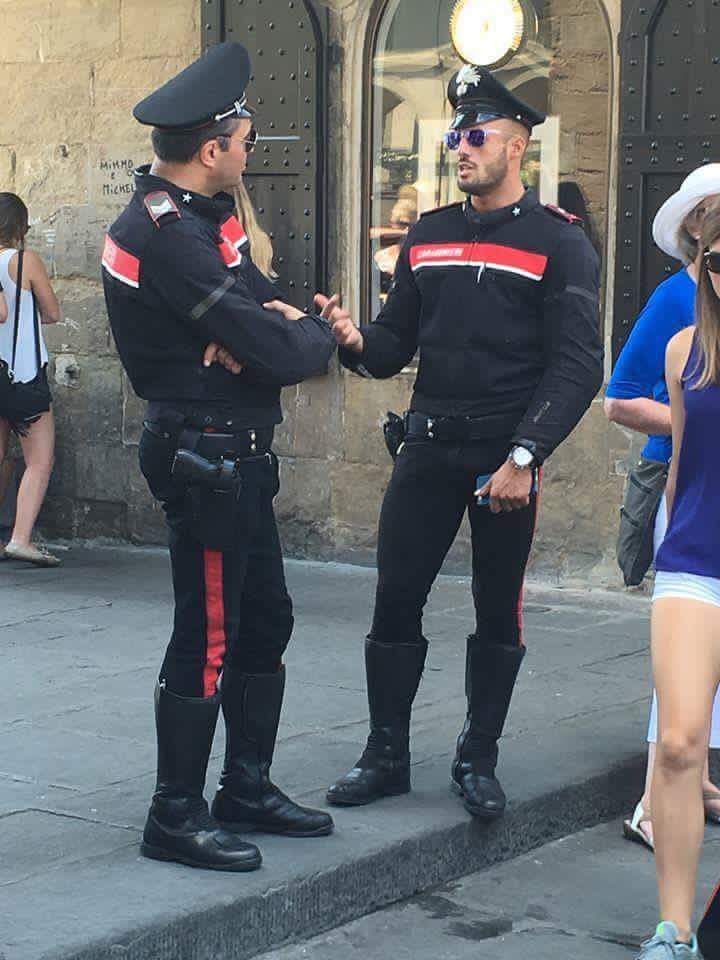In a bustling pedestrian street of a European cityscape, two men stand at the center of the image dressed in striking black and red police uniforms. Each uniform features black pants adorned with a vivid red stripe down the sides, paired with black motorcycle boots that nearly reach their knees. Their black jackets also sport a red stripe across the chest, accented with some unreadable white lettering. Both men wear dark sunglasses and black caps with an emblem on the front, and are armed with pistols at their waists. One officer, who has a watch on his left wrist and a phone in hand, stands with his hand out as he talks to the other, who listens with his arms crossed. Surrounding them, several women, likely tourists, partially frame the scene; they are dressed in summer attire including shorts and sunglasses. To the right, a woman in a blue shirt and short white shorts is walking, accompanied by another woman wearing a white hat and blue shirt. A third woman in a white top and black short shorts can be seen in the back left, looking at a stone wall. The backdrop reveals a stone building with a large window framed by black shutters, adding to the picturesque European city atmosphere.